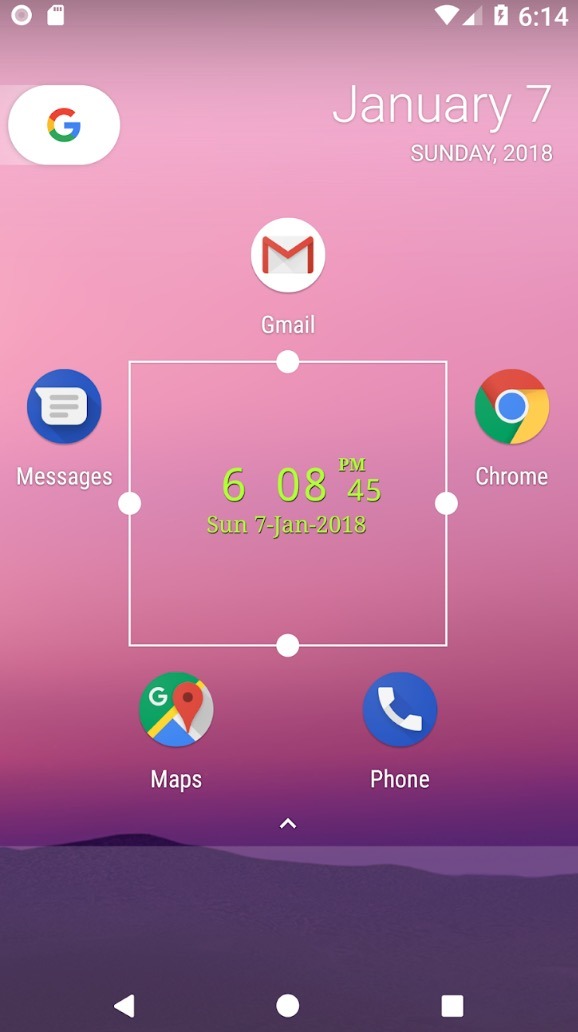The image is a vertically oriented screenshot of a smartphone display, featuring a sleek background with a gradient effect transitioning from various shades of pink and purple to a sharp gray at the bottom, giving it a multidimensional feel. 

In the upper left and right corners, there are several icons. Notably, the upper right includes a partially filled triangle facing down and a battery icon indicating it's charging at 6:14 PM. Alongside, the Google logo is visible on the left side of the screen, with "January 7th," "Sunday," and "2018" displayed on the right.

Centrally located on the screen is a white square surrounded by circular icons with their respective names above them. At the top, there is the Gmail icon with the label "Gmail." Nearby is the Messages icon labeled "Messages." Below are the Maps and Phone icons, each inside small white circles. To the right is another white circle containing the Chrome icon.

The time "6:08 PM 45 seconds," along with the date "Sunday, the 7th of January 2018," is clearly displayed in the center of the screen. Finally, at the bottom, navigation icons are visible: a triangle pointing left, a filled-in circle, and a filled-in square on the right.